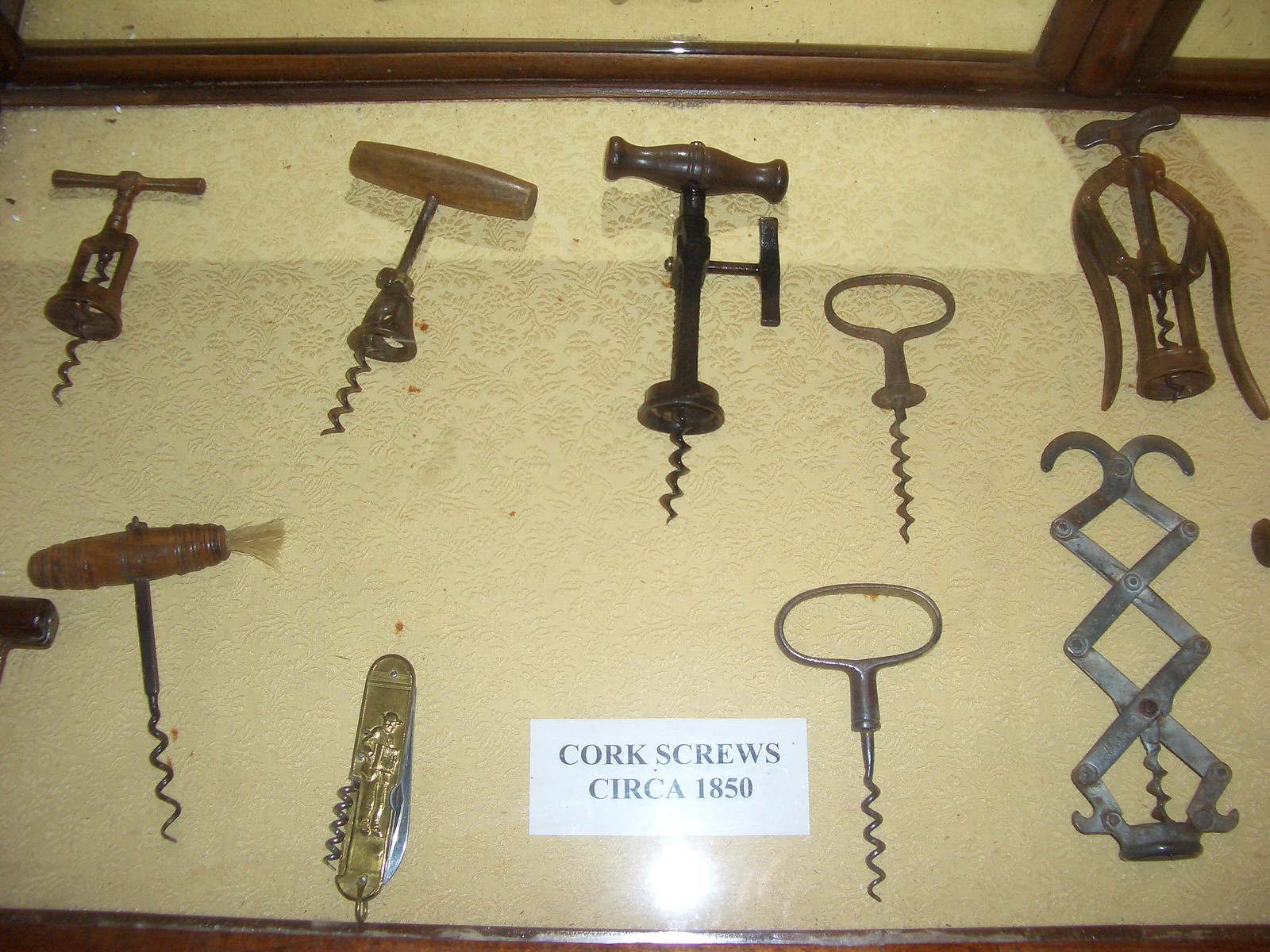The color photograph captures a display case in a museum, showcasing a collection of antique corkscrews circa 1850. The case features a dark wood frame and a glass top, beneath which lies a white label with black text reading "Corkscrews circa 1850". The display is illuminated by a flash, casting a bright highlight at the bottom center of the image, and the overall photo has a light yellow or sepia tint.

Inside the case, against a beige cloth background, roughly ten corkscrews are meticulously arranged. These corkscrews are primarily composed of metal and wood, exhibiting signs of aging such as rust. Each corkscrew’s handle varies in color and material: some are made of dark wood, possibly ebony, while others range from lighter to medium brown. Notably, there is a corkscrew with a metallic handle in a zigzag pattern located in the lower right-hand corner, and a distinctive gold corkscrew, resembling a part of a pocket knife, situated in the lower left-hand corner.

This detailed and diverse range of vintage corkscrews highlights the craftsmanship of the mid-19th century, offering an intriguing glimpse into historical tools used for opening wine bottles.